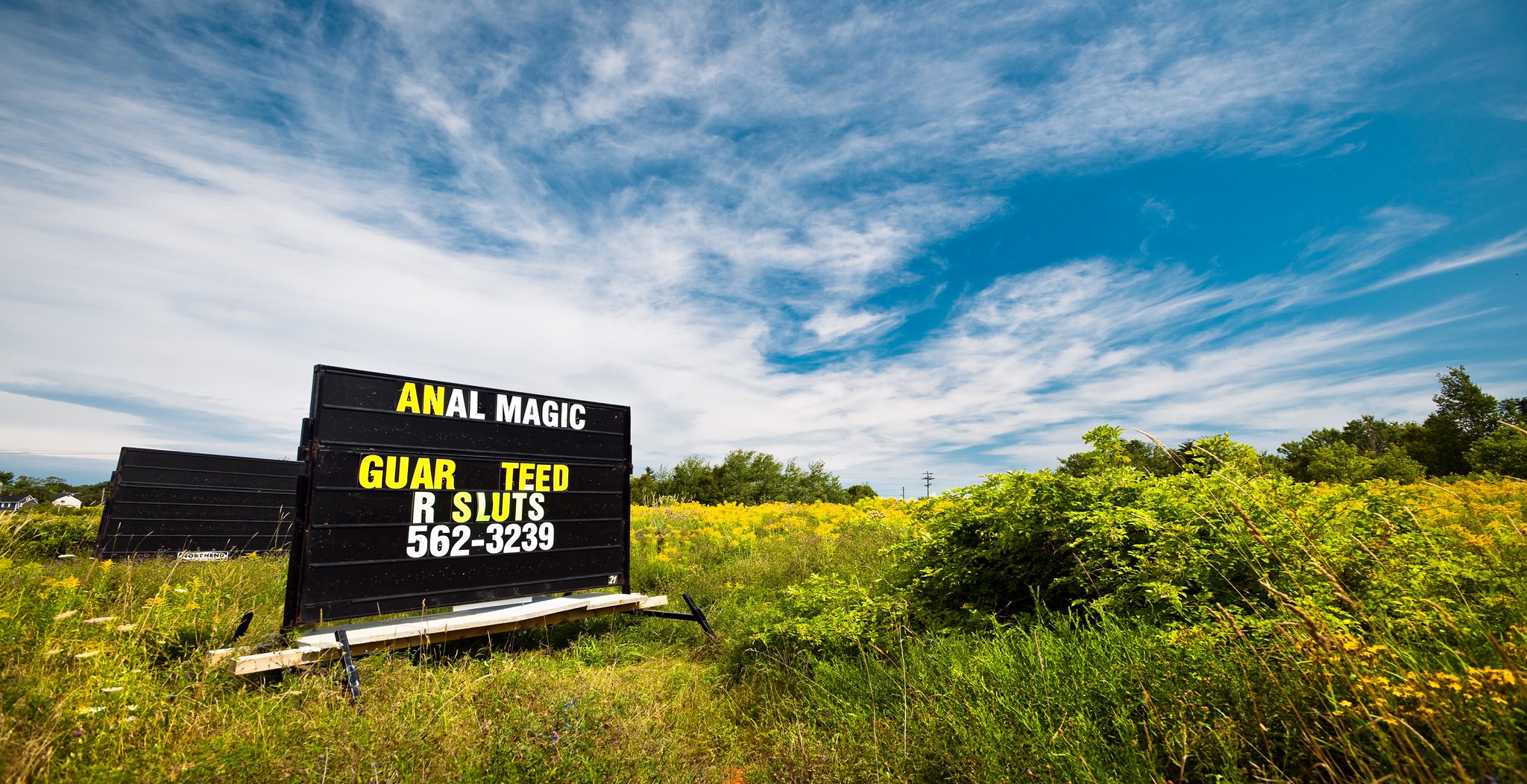The image captures a sunny day with a vibrant blue sky dotted by sparse white clouds. The scene is dominated by an open yard filled with tall grass and dotted with flowers, predominantly yellow. Positioned centrally, but slightly to the left, stands a signboard perched on a white wooden stand. This main sign, which features a mixture of orange and yellow text, reads "ANAL Y METRIC GUARANTEED RESULTS," along with the phone number "562-3239." The sign also has some partially obscured letters. In the background, a second sign is visible, though it appears either blank or with its back turned to the camera. There are other minor details including a visible power line stretching across the blue sky and some distant white houses with black roofs to the left side of the image. This well-lit scene suggests a clear, bright day, emphasizing both the natural beauty of the area and the handcrafted signs.